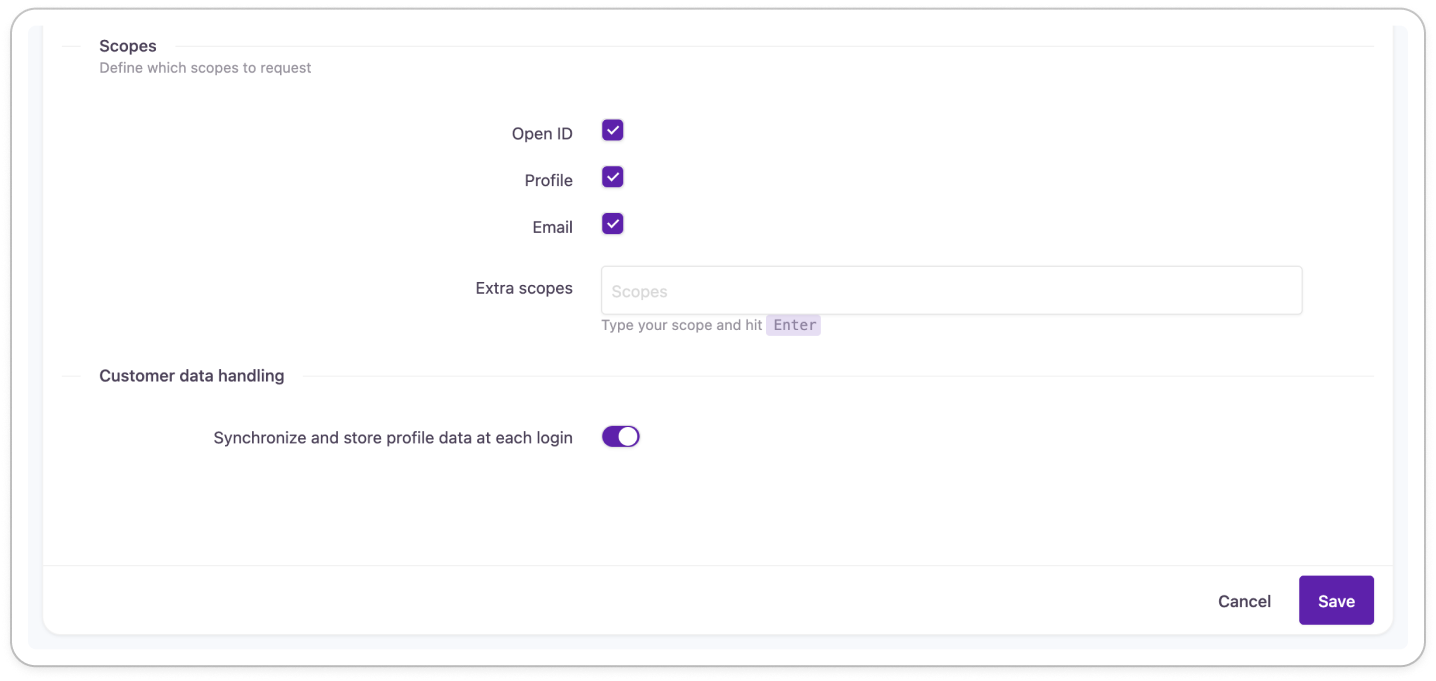The image depicts a section of a user interface (UI) with a focus on the bottom portion of a screen, against a predominantly white background. The content appears to be user settings related to OAuth scopes. The header in the upper left corner is labeled "Scopes," with a subheading "Define which scopes to request."

Three scopes are listed, each with a purple checkmark:

1. **OpenID**
2. **Profile**
3. **Email**

Below these, there is an "Extra scopes" section featuring a text input field marked with the placeholder "Scopes." It prompts the user to type desired scopes and press Enter.

Further down, there is a section labeled "Customer data handling," accompanied by a description: "Synchronize and store profile data at each login." A toggle switch next to this description is set to the "on" position, indicated by its purple color.

In the bottom right corner, there are two buttons: "Cancel" in black text and "Save" in purple text on a white background. The entire interface is framed by a subtle gray border, distinguishing the white content box from the background.